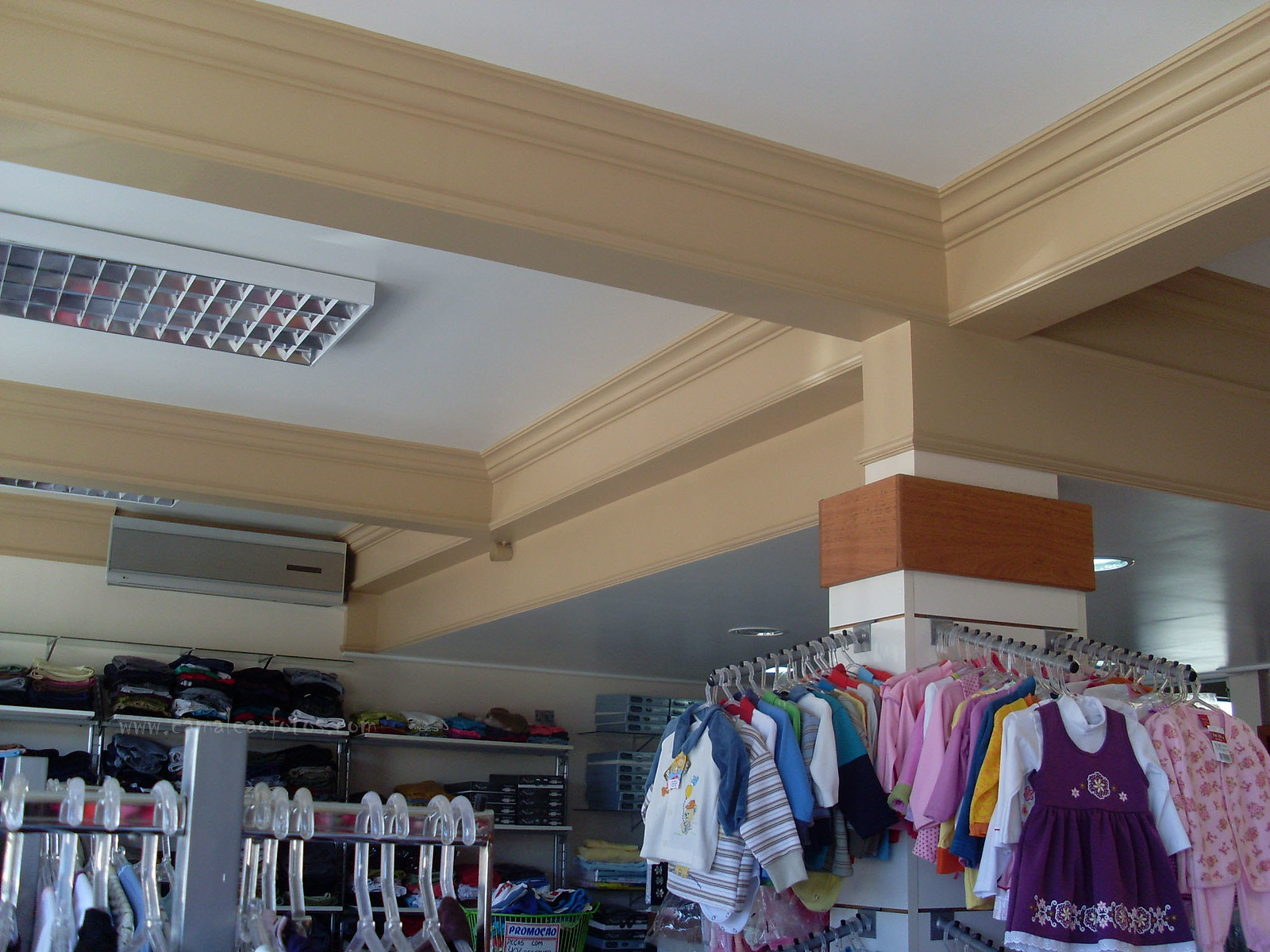The image depicts the interior of a modern children's clothing store, captured from a slightly elevated angle. The ceiling is white with prominently thick, tan wooden beams running horizontally across it, adding a touch of elegance to the space. Stylish recessed lighting is installed, complemented by rectangular fluorescent fixtures that illuminate the area brightly. There is also a new air conditioning unit positioned in a corner, ensuring the store remains cool and comfortable.

The store is freshly painted and meticulously organized. Along the walls, there are shelves neatly stacked with colorful clothing items, showcasing boys' clothes in shades of blue, green, and red on the left side and girls' clothes in lighter colors and pinks on the right. Embellishing the walls are T-shaped racks, extending from square supports, adorned with clear plastic hangers. Although the specific outfits are not visible, the arrangement suggests they are ready for easy browsing.

In the background, additional shelving can be seen, filled with folded clothing items, adding to the abundance of options available in the store. The overall ambiance of the store is clean, vibrant, and inviting, making it an ideal shopping destination for children's apparel.